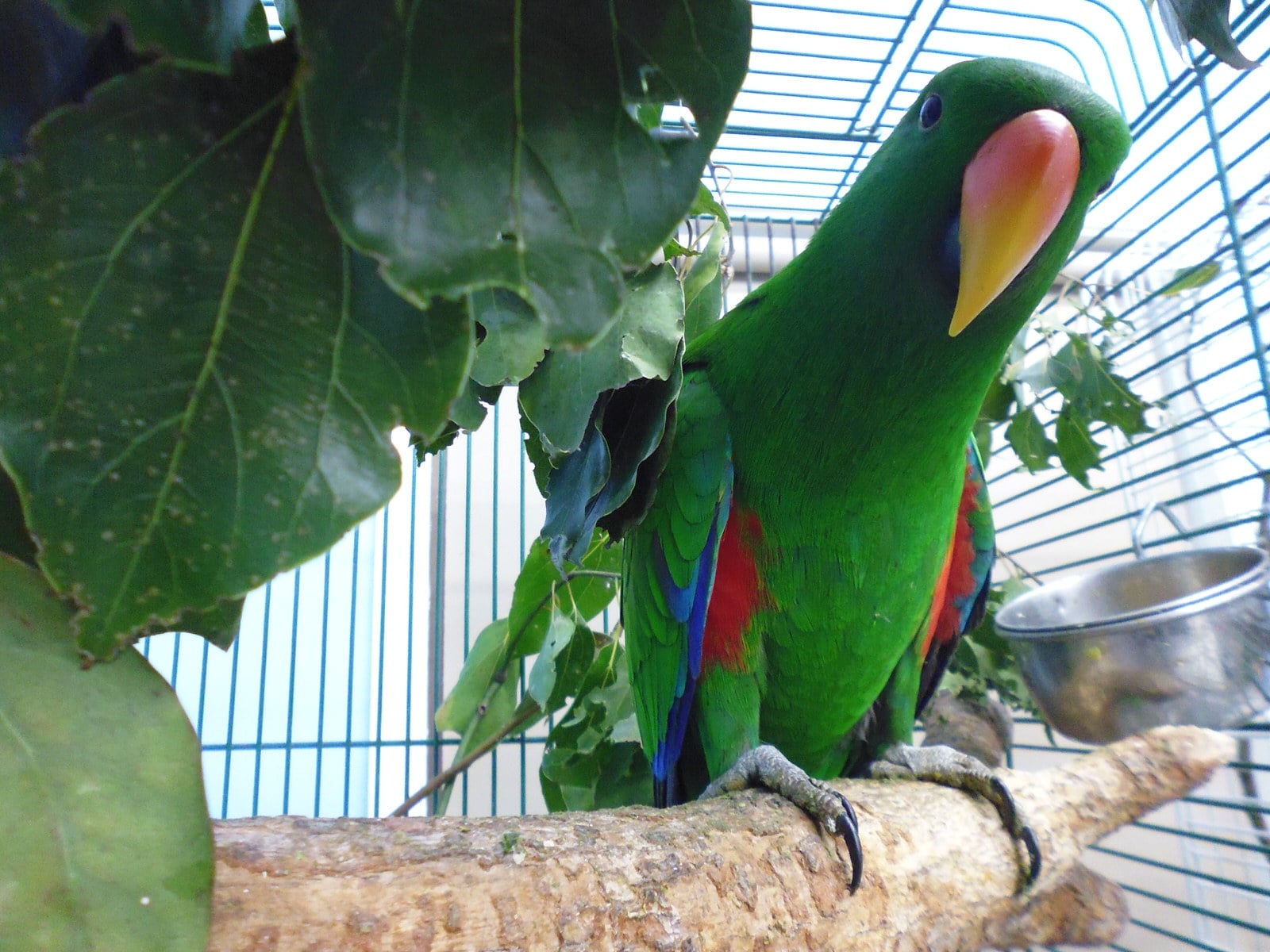The image captures a vibrant green parrot with an intricately colored beak that transitions from orange at the top to yellow at the tip. The parrot, highlighted with blue and red accents on its wings and legs, is standing on a wooden branch inside a steel wire cage. It gazes directly at the camera with its head slightly tilted, exuding a sense of curiosity and charm. The cage is adorned with lush green foliage on the left, providing a natural backdrop, while a small silver metal feed tray or water cup is visible to the right. The overall composition emphasizes the parrot's colorful plumage and lively demeanor within its verdant enclosure.